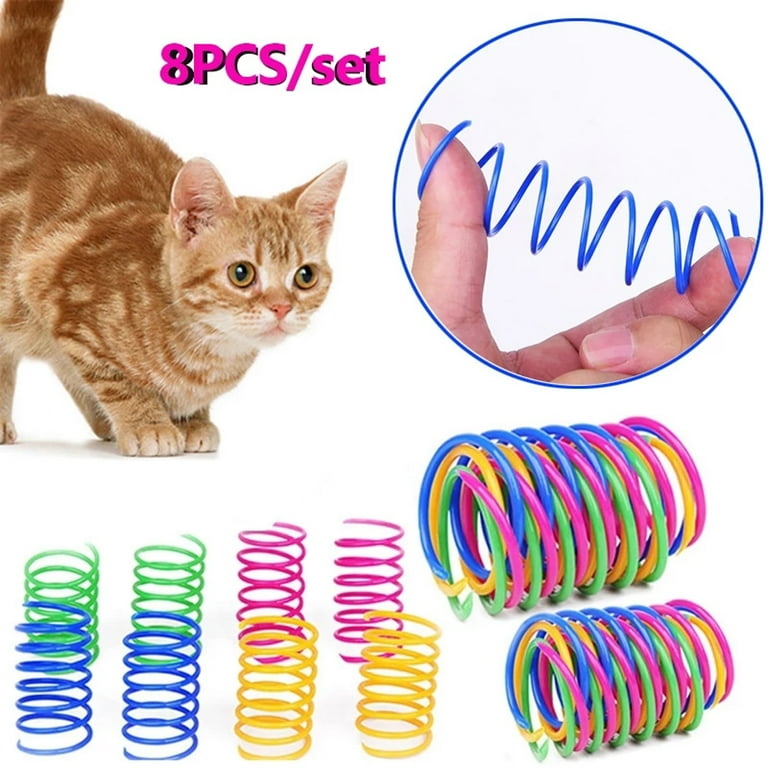This square-shaped image, without a border, predominantly features an advertisement for an 8-piece set of multicolored spring toys designed for cats. In the upper left-hand corner, there's an orange and brown cat with cute golden-black eyes, a pink nose, and pointy ears. The cat's two front paws are positioned closely together as it gazes intently at the toys. Above its head, in purple text, it reads "Eight pieces per set." On the upper right side of the image, there is a large blue-outlined circle showing a person's hand manipulating a small blue coiled toy between their thumb and index finger, demonstrating the toy's flexibility. Below, in the lower-right corner, several coiled toys in various colors – two blue, two green, two purple, and two yellow – are depicted, some standing vertically and others lying horizontally, illustrating the different ways they can be arranged and combined. The coiled toys appear interlocked and squished together, showcasing their versatility and appeal as playful objects for pets.